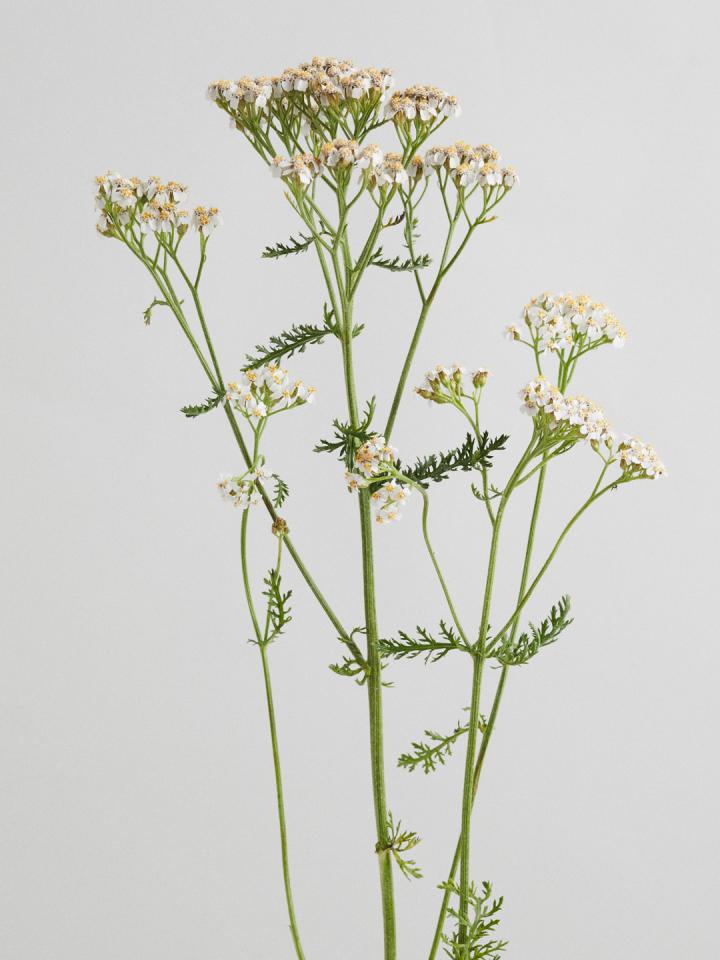The image features a delicate arrangement of flowers set against a gray background. Central to the composition are slender, green stems that extend vertically from the bottom almost to the top of the frame, flanking both the left and right sides. Each stem branches off into smaller stems adorned with green leaves. At the pinnacle of these stems sit tiny, bulb-shaped flowers that are predominantly white with subtle hints of orange and yellow at their centers. The simplicity and elegance of the flowers are highlighted by the gray backdrop, allowing the intricate details of the thin, green stems and the delicate, white blossoms to stand out prominently.